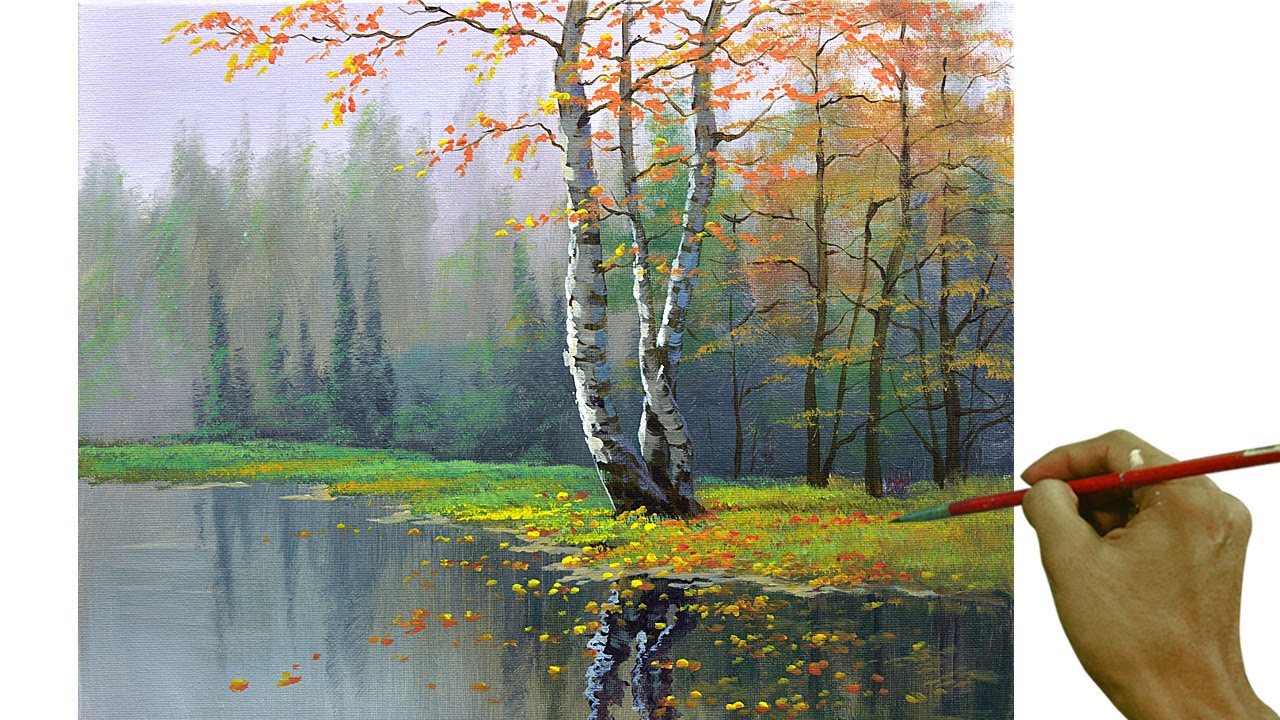The image appears to depict an autumnal landscape, likely created as a paint-by-number or watercolor painting. It showcases a serene outdoor scene, featuring the bank of a lake or river with grayish-blue water that reflects the surrounding trees and foliage. In the foreground, a prominent birch tree with vivid yellow and orange leaves stands out, its reflection mirrored in the water below. Scattered around the grassy shore are fallen leaves in shades of orange and yellow, intermingling with the darker green grass and small pine bushes. Further back, a mix of thin brown trees and additional birch trees add depth to the scene, their autumn-colored leaves contrasting with the greenery. On the right side of the image, a hand holding a red paintbrush is seen, suggesting an artist actively working on the painting. The background hints at a hazy, cloudy day with a bluish-gray sky, adding to the tranquil autumn atmosphere.